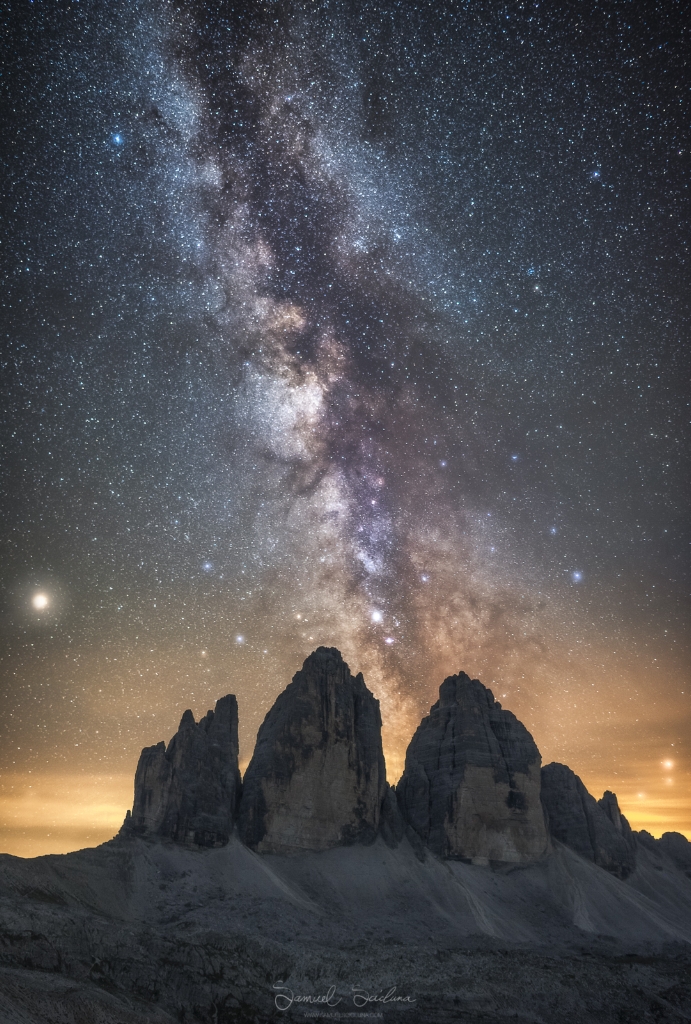A stunning photograph by Samuel, possibly taken in a desert region near Sun City, showcases a breathtaking night sky filled with a dazzling display of stars. The sky, occupying the upper three-quarters of this portrait-oriented image, features a vibrant Milky Way running vertically with visible nebulae, gas clouds, and a dense array of stars in varying sizes and colors. The horizon seems to catch the last rays of a setting sun, with an orange glow hinting at a long exposure capture. Below this celestial panorama, the lower quarter of the image depicts rugged, jagged mountain formations surrounded by smoother, sloping terrains and sparse desert vegetation, creating a stark but beautiful foreground to the mesmerizing night sky above.